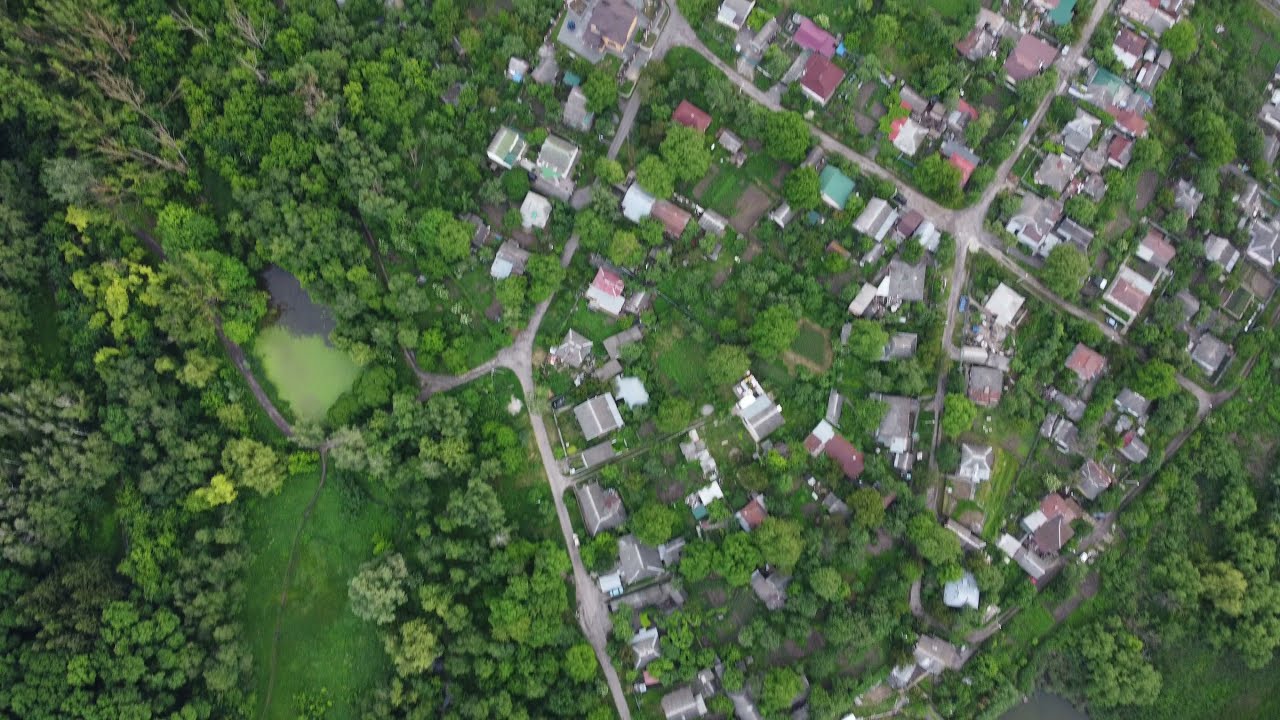This aerial image, likely captured by a drone or satellite, showcases a suburban town sprawling predominantly in the right two-thirds of the frame. The town is characterized by a variety of colorful rooftops, including green, red, and gray, and the homes are somewhat scattered amidst an abundant landscape of trees, bushes, and grassy patches. The left side of the image starkly contrasts this suburban layout with a lush, uninterrupted expanse of forest, teeming with greenery. This side of the frame might also feature a small lake, though its presence isn't entirely clear. Overall, the image highlights a verdant, semi-wooded residential area with a mix of houses and ample green spaces, crisscrossed by a network of small roads.